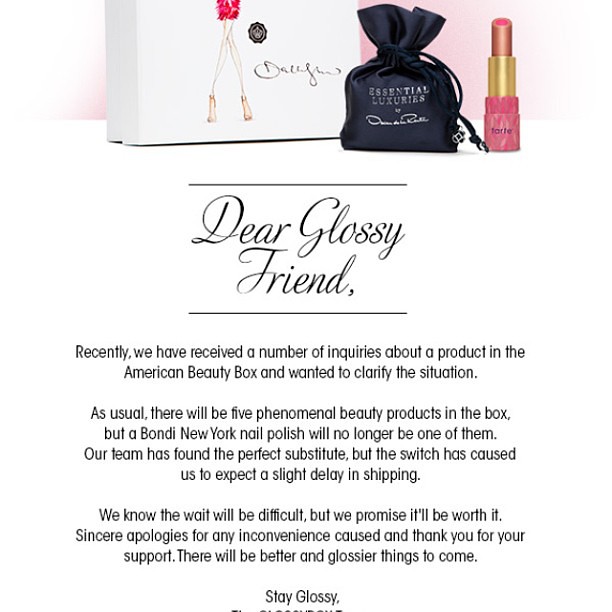The image appears to be a scanned advertisement or announcement printed on a piece of paper. At the top, there is a prominent, elegantly cursive heading that reads "Dear Glossy Friend." Just below this heading to the left, there's a picture of a small, black silk bag inscribed with "Essential Luxuries" in off-white cursive. To the right of the bag, there's an upscale pink lipstick with a gold base, branded as "TARTE," and beside it, a white box showing an illustration of very slender women's legs.

Below this cluster of images, a message is written in a combination of cursive and regular fonts. It starts with the cursive script "Dear Glossy Friend," followed by non-cursive text: "Recently we've received a number of inquiries about a product in the American Beauty box and wanted to clarify the situation." The message continues to explain that while five phenomenal beauty products will still be included in the box, the Bondi New York nail polish will no longer be one of them. A perfect substitute has been found, but this switch will cause a slight delay in shipping. The message concludes with, "We know the wait will be difficult, but we promise it will be worth it. Sincere apologies for any inconvenience caused and thank you for your support. There will be better and glossier things to come." At the very bottom, in regular print, it says "Stay Glossy."